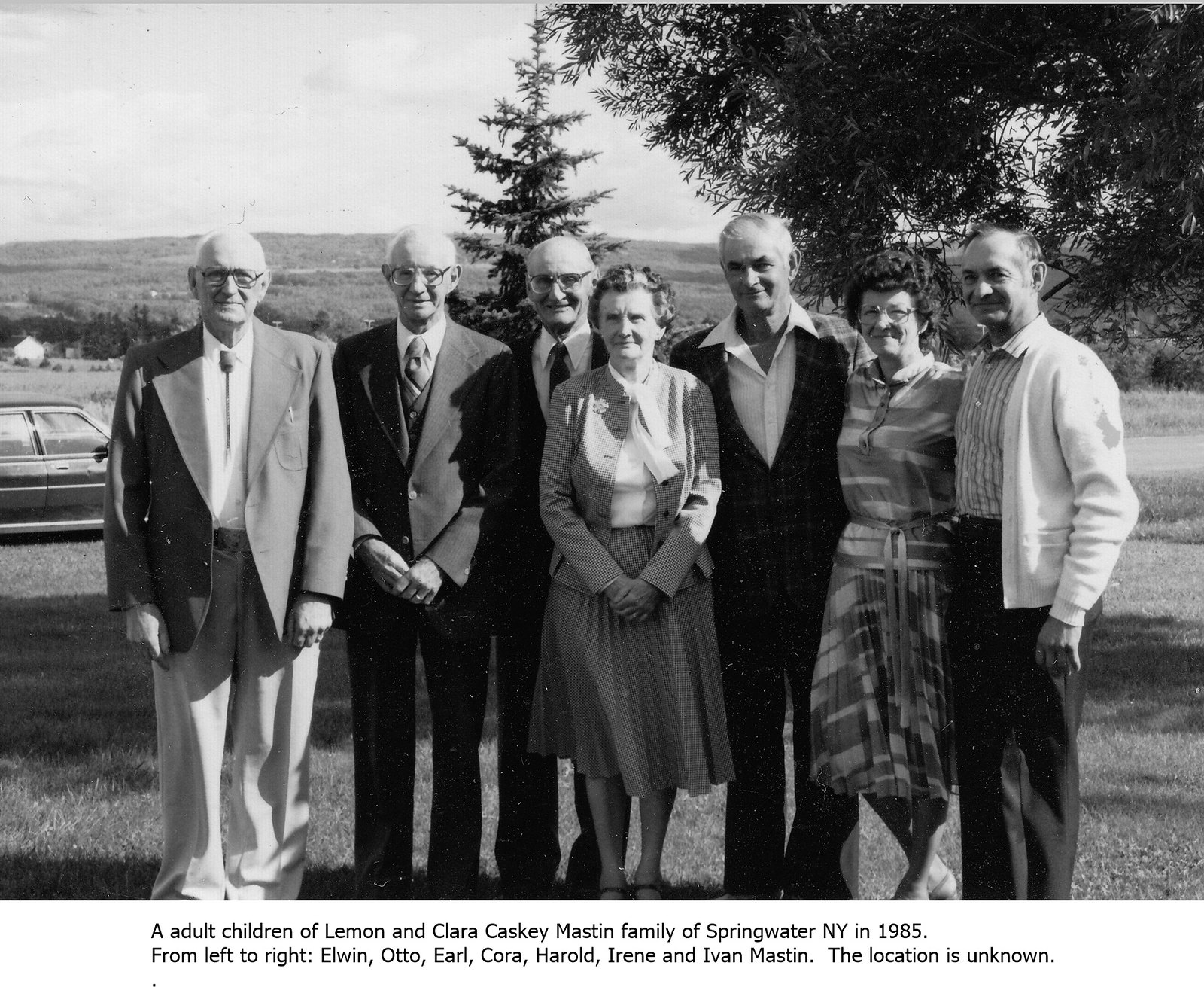A black-and-white portrait photograph from 1985 captures the adult children of Lemon and Clara Caskey, identified as the Masten family from Springwater, New York. This familial gathering presents seven Caucasian individuals. From left to right, they are named Elwin, Otto, Earl, Cora, Harold, Irene, and Ivan Mastin. The men exhibit a range of formal attire: Elwin wears a Texas bow tie with his blazer, Otto dons a traditional suit and tie, while Earl is suited and slightly obstructed by Cora, who stands in front. Cora is dressed in a sweater and skirt combination. Harold sports a white shirt with a vest, and beside him stands Irene in a patterned dress and glasses. Lastly, Ivan wears a light-colored sweater over a button-down shirt paired with dark slacks. The entire group poses outdoors against a backdrop of trees, with a distant car and countryside barely visible. Though the clothing styles appear reminiscent of the 1960s, the text beneath the photograph clearly states it was taken in 1985. The exact location remains unknown.